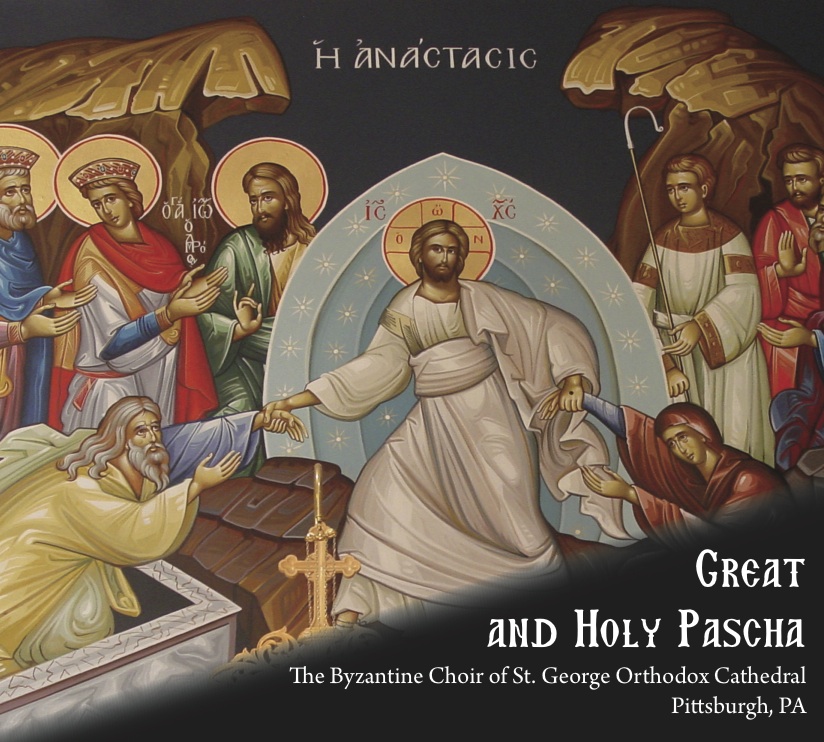The image is a detailed religious painting advertising "Great and Holy P.A.S.C.H.A.," credited to The Byzantine Choir of St. George Orthodox Cathedral, Pittsburgh, PA. The focal point is Jesus, centrally positioned against a blue arch, surrounded by His apostles adorned in vivid robes of various colors including white, green, red, yellow, and blue. The background appears dark, possibly black, with elements suggesting palm trees. Jesus is depicted holding hands with two men, one in a yellow robe on His left and another in a red robe on His right. Surrounding Him are several other figures, some of whom wear crowns, and one is seen holding a staff. Text in an unreadable script is present at the top of the image. The composition is vibrant and meticulously detailed, capturing a moment of reverence with figures seemingly reaching towards Jesus in adoration.